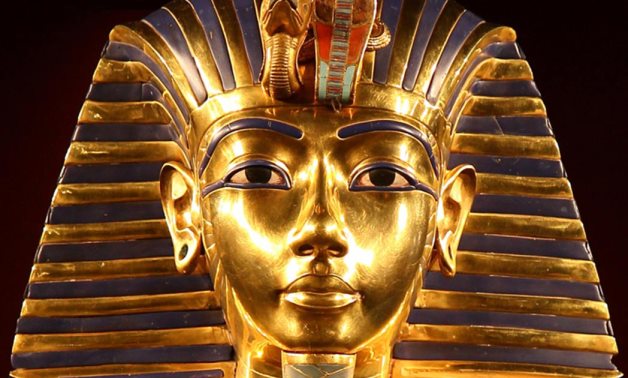This image depicts the intricately designed golden funeral mask of an ancient Egyptian pharaoh, likely King Tutankhamun. The mask is predominantly painted with metallic gold and features striking blue stripes on the headdress, which extends from slightly below the chin to the edge on either side but is cropped at the top of the image. Central to the headpiece is an elaborate depiction of what appears to be two intertwined snakes—a cobra and possibly an asp—with the cobra adorned with red and teal embellishments. The pharaoh’s face is framed by navy blue eyebrows and elaborately painted eyeliner that wings out from his eyes, emphasizing his piercing gaze. His ears are noticeably pierced. The detailed craftsmanship of the mask against a solid black background accentuates its majestic and somber presence.